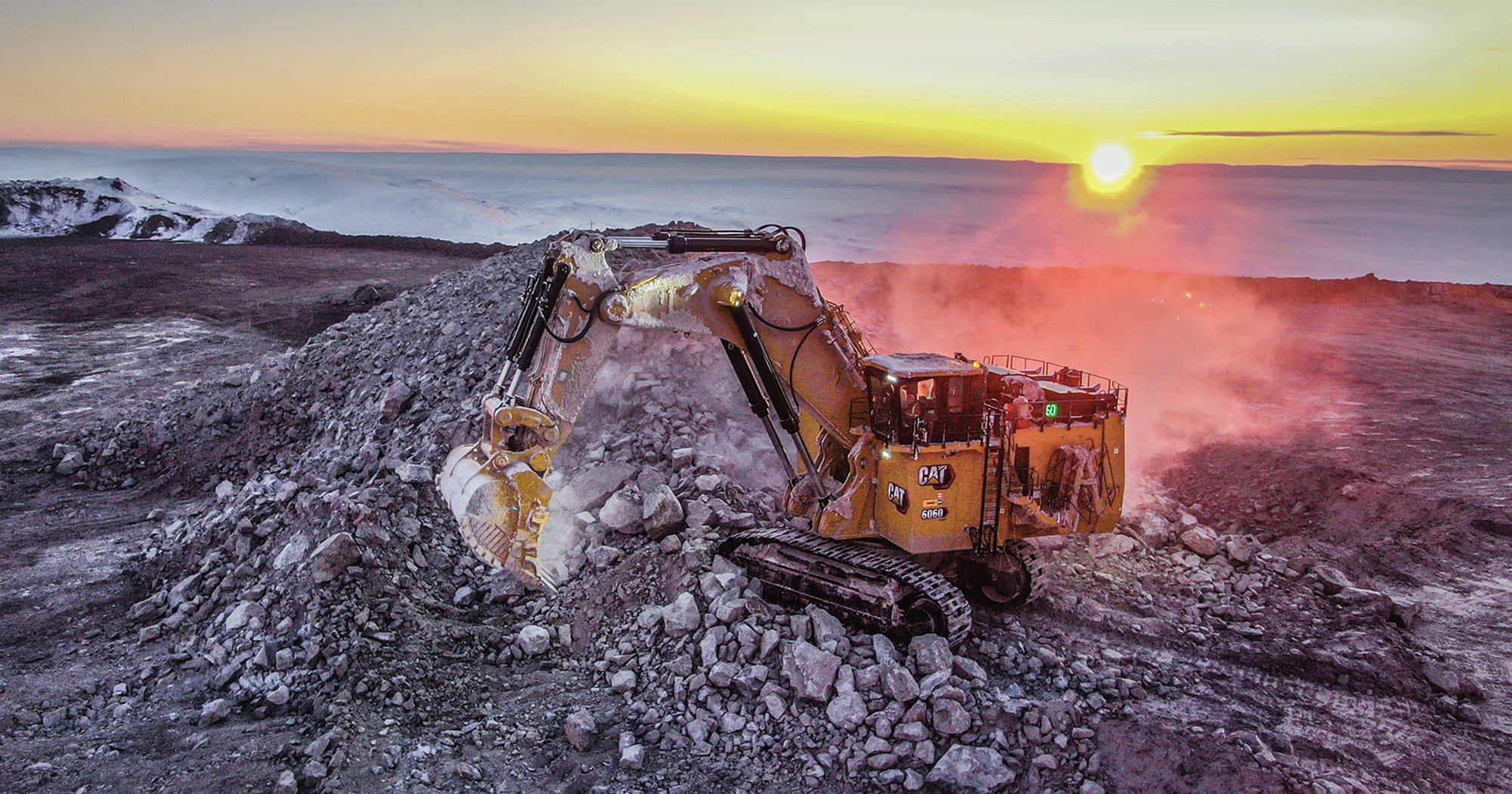The image depicts a coastal construction site at sunset, where a bright yellow excavator with prominent CAT logos is actively digging and moving light gray rocks. The machine's large claw is poised to scoop up the rocky terrain, and dust can be seen billowing up from the work. The surrounding landscape consists of mounds of dirt and granite gray rocks, indicative of a rock quarry. Far across the horizon, the sun is setting into a body of water, casting a golden yellow and off-white hue across the sky. The tranquil sea and the ball of the setting sun create a contrasting backdrop to the busy scene of excavation in the foreground.